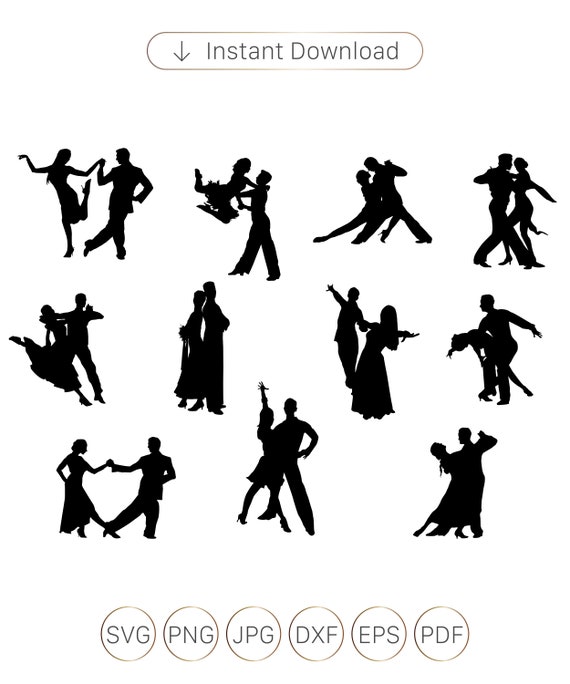This is a clipart image depicting 11 different silhouettes of couples in various dance poses against a transparent background. At the top of the image, there is a thin, long gray rectangle (or oval) with a down arrow and the phrase "Instant Download" written in gray, indicating it is available for download. The bottom of the image features six gray-outlined circles, each labeled with different file formats: SVG, PNG, JPG, DXF, EPS, and PDF. The couples, possibly a man and a woman, are shown engaging in professional dance moves, with one notable pair in the bottom left corner forming a heart-like shape as they pull apart while their arms and legs cross.